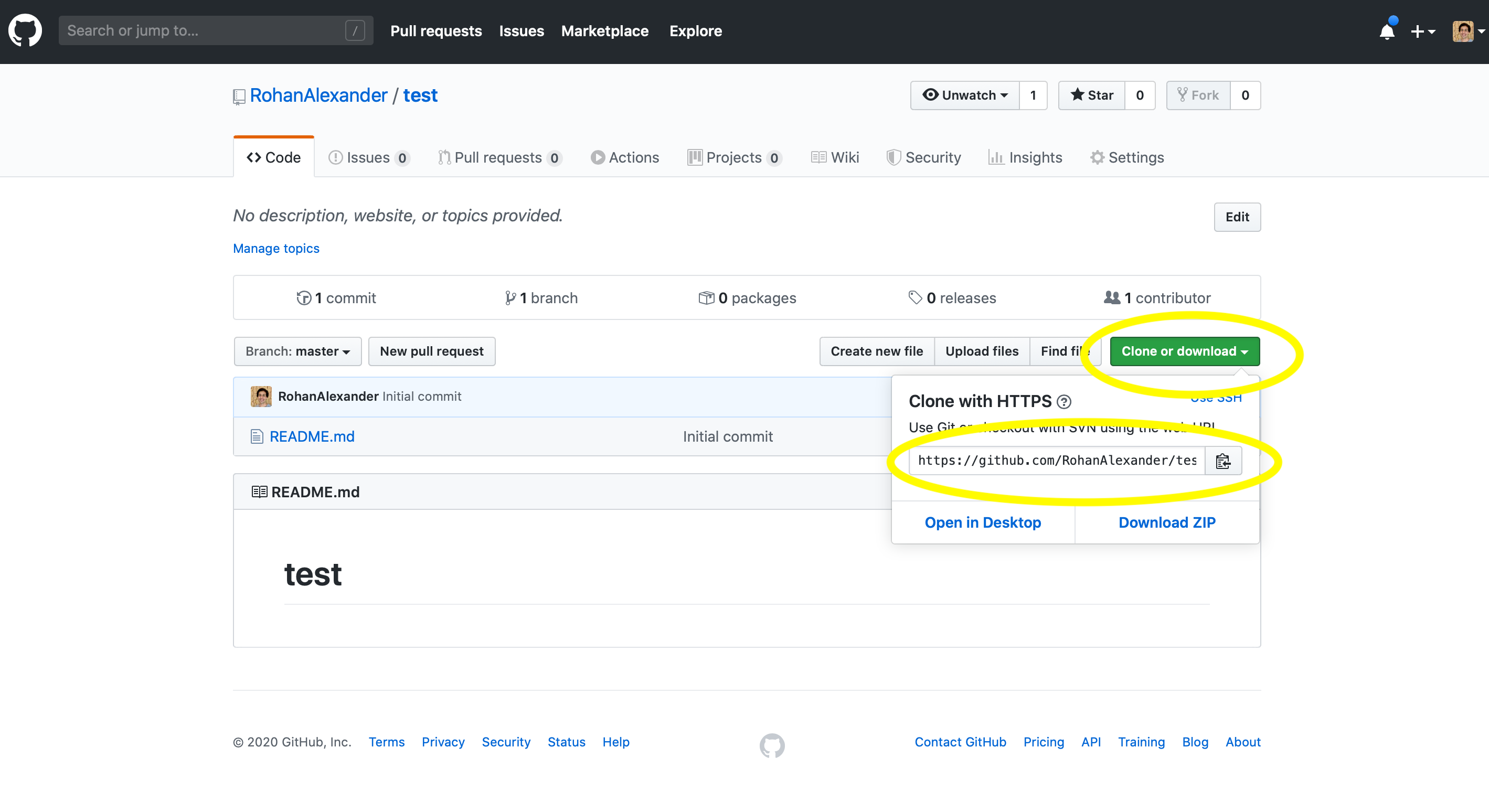The top five to ten percent of the screen features a black horizontal bar. In the top-left corner, there's a cat icon resembling a silhouette set against a white circle. Directly to its right is a search bar labeled "Search or jump to..." Further right, there's white text that reads "Pull requests," "Issues," "Marketplace," and "Explore." 

On the top-right side of the bar, there is a white bell icon with a blue dot indicating notifications, followed by a plus icon with a dropdown arrow and a profile icon also with a dropdown arrow. Adjacent to these icons, there is blue text divided by a gray slash, which precedes three buttons. Each button has a white square next to it displaying numbers; the sequence is "1," "0," and "0."

Below the black bar, there are nine tab options, with the first tab selected. This tab is highlighted by an orange horizontal bar above it and is labeled "Code." Beside it to the left is a gray backslash symbol. Underneath the tab area, on the far right, there is a green button encircled by a yellow oval, and an HTTPS link similarly outlined by the same yellow oval.